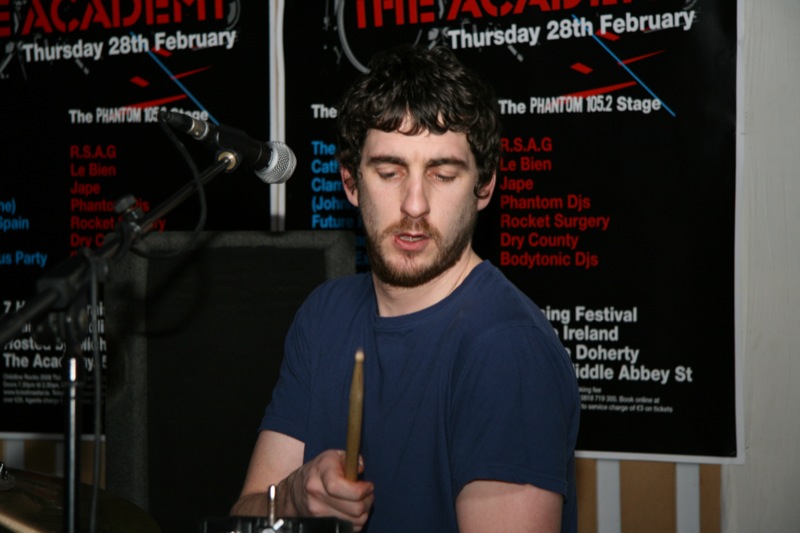The photograph captures a man mid-performance, playing the drums. With dark curly hair, a short beard, and fair skin, he is focused intently on his instrument, looking down without making direct eye contact with the viewer. Clad in a navy blue t-shirt, he confidently grips a wooden drumstick in one hand. Positioned beside him is a silver and black microphone on a stand, and a prominent black speaker looms in the background. Scattered around his drum kit are glimpses of other instruments, including the neck of a guitar, suggesting his versatility.

Two large identical posters dominate the backdrop, partially obscured by the man. They bear red text at the top, "Academy" followed by "Thursday, 28th February" in white text. Below, a list of performances in various colored texts mentions "RSAG," "Labine," "JAPE," "Phantom DJs," "Rocket Surgery," "Dry County," and "Bodytronic DJs." Further obscured details in white text include "Festival Ireland," and "Doherty, Abbey Street." Despite the partial obstructions, the scene vividly conveys the atmosphere of an active and diverse musical event.